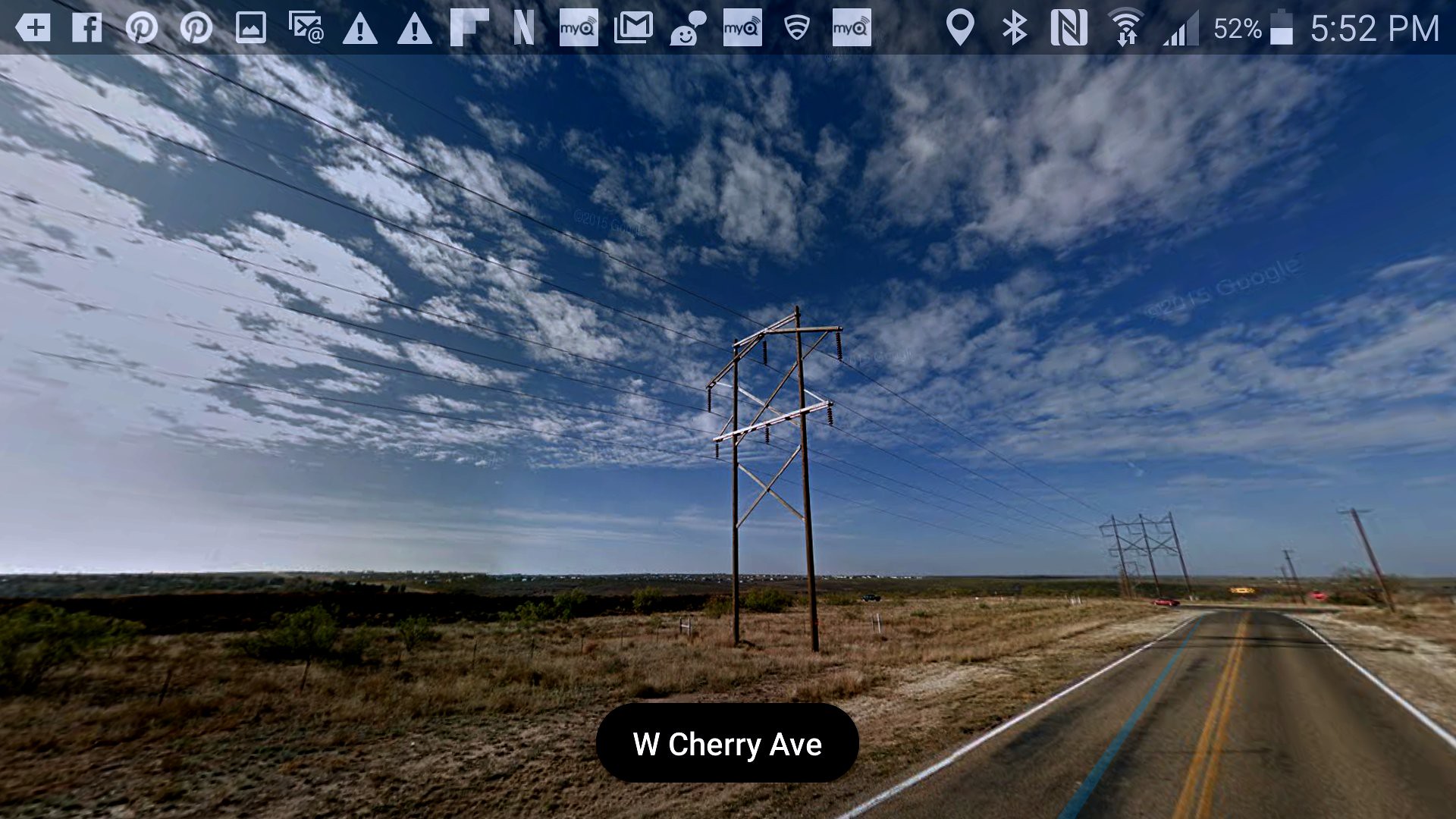This is a screenshot taken from a smartphone, evident by the status bar at the top that includes various indicators: a 52% battery life, time displayed as 5:52 PM, signal strength with three bars, Bluetooth connectivity, and several notification icons for apps like Facebook, Pinterest, email, and general caution alerts. The primary content of the screenshot is a Google Maps Street View image captioned "West Cherry Avenue" at the bottom. The image depicts a long, empty road with a solid yellow line in the center and a blue line on the left side. On the left side of the road are brown fields and power lines, while on the right side, more power lines are visible in the distance. The sky is a vibrant blue filled with scattered clouds, giving an open and expansive feel to the scene. No buildings are present, suggesting a remote area.